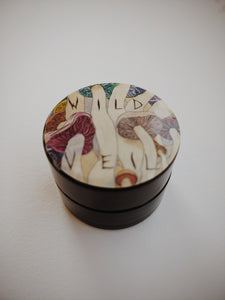This photograph depicts a small, black metal canister with a screw-off top, positioned on a white surface. The top of the canister features a vibrant, hand-drawn illustration of various colorful mushrooms, some of which are red with thick stalks, while others are blue, orange, pink, brown, and even green. The mushrooms are seen from an upward viewpoint, creating an artistic and whimsical effect. Prominently displayed on the top of the canister is the phrase "Wild Vale," written in stylistic black text that appears as part of the design itself. The canister's bottom half appears slightly smaller, likely due to the angle of the photograph. This detailed and intriguing design suggests that it might be an artisanal product container, possibly for wild mushrooms or another specialty item.